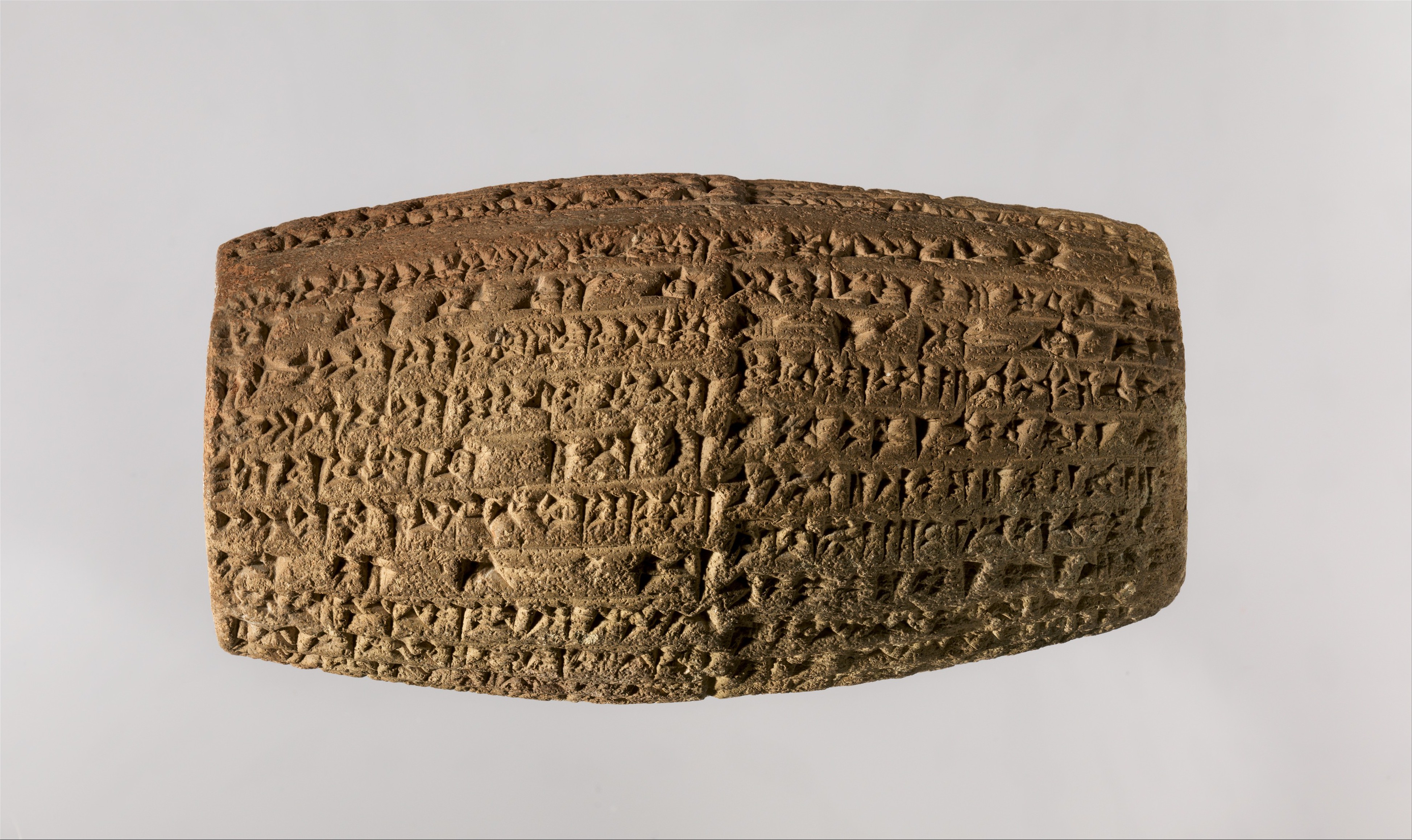This image features an ancient-looking tablet made from a golden dark stone, set against a grey background. The object is roughly rectangular and sizeable, resembling an artifact one might find in a museum or on a history channel. The tablet is divided into two distinct sections, separated by a central ridge that runs vertically like the spine of a book. Each side of the tablet contains a series of 6 to 8 horizontal lines filled with intricate characters, symbols, or hieroglyphics that are hard to decipher. The stone surface is detailed with numerous indents and engravings, suggesting a rich and possibly historical significance.